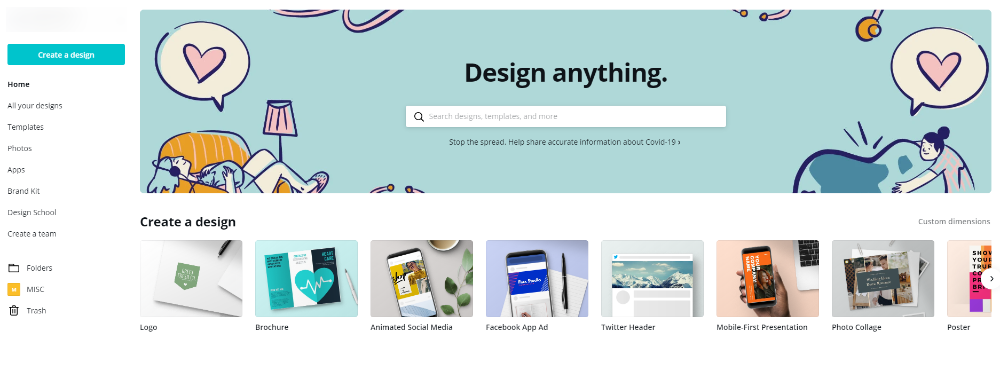The image depicts a webpage from a design-oriented site. At the top of the site is a main banner with the text "Design Anything" center-justified. Below the banner is a search bar, also center-justified. Beneath the search bar, there's a smaller font text that reads, "To stop the spread, help share accurate information about COVID-19." These elements are framed within a light green banner. Within this banner, there is an illustration: on the left, a person is lying sideways on a chair, wearing headphones. On the right, another figure appears to be embracing a globe-like symbol. To the left side of the page, there is a vertical menu. The menu items include "Create a Design" at the top, followed by "Home," and "All Your Designs."